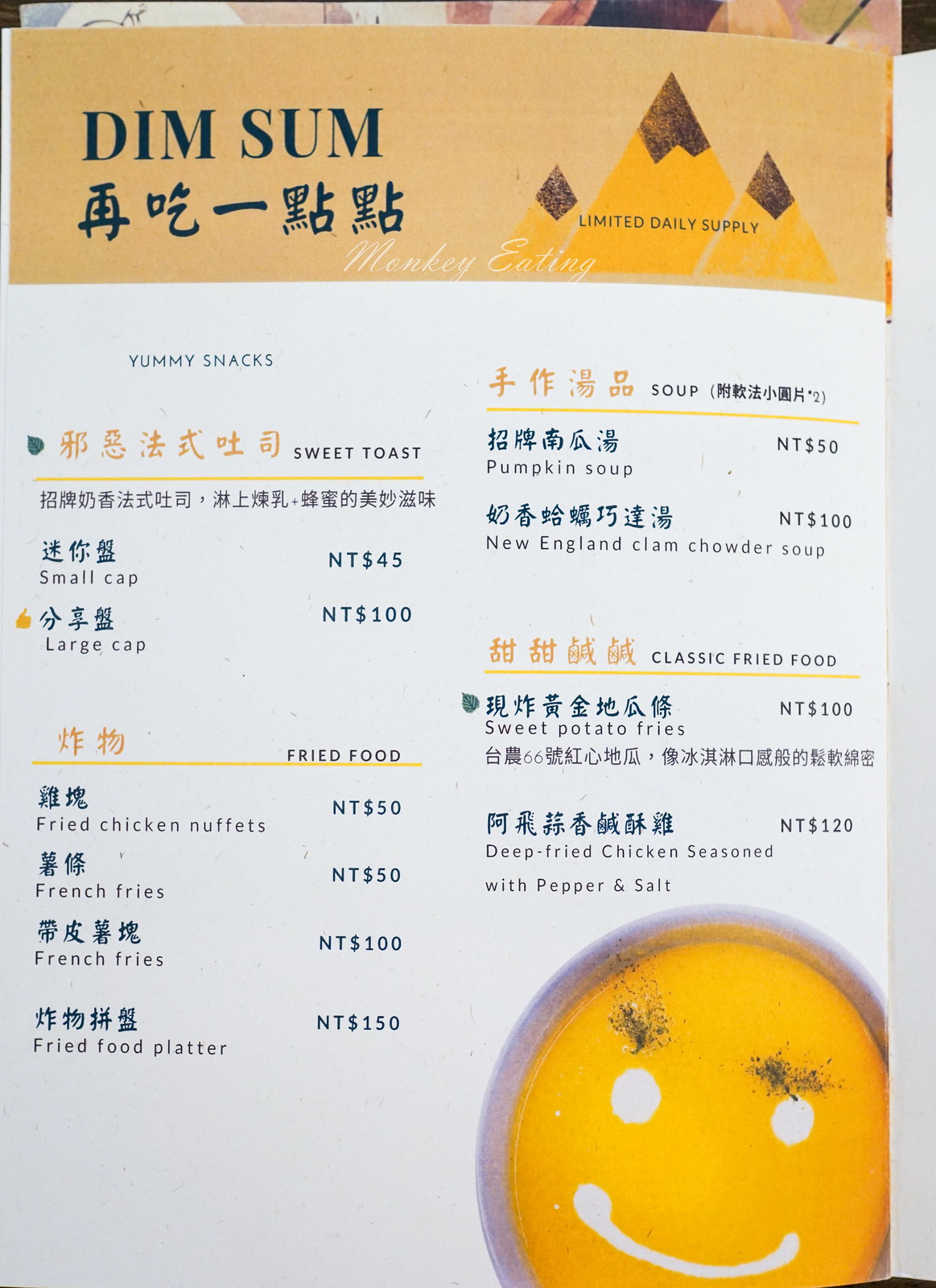This image displays a detailed menu from what appears to be a Chinese restaurant, prominently featuring the title "Dim Sum" in an orange section at the top. Below the title, there are kanji characters, indicating the restaurant's cultural heritage. Adjacent to the "Dim Sum" heading, three stylized orange mountains with darker brown tops accompany the text "Limited Daily Supply."

Beneath this, the menu lists various food items, starting with a section titled "Yummy Snacks," which includes:

- Sweet Toast: Small (NT 45), Large (NT 100)

Following "Yummy Snacks," the menu transitions to a "Fried Food" section, offering:

- Not Enough: NT 50
- French Fries: NT 50
- French Fries (another type): NT 100
- Fried Food Platter: NT 150

In the right column, the "Soup" selections are:

- Pumpkin Soup: NT 50
- New England Clam Chowder Soup: NT 100

Further down, the "Classic Fried Food" section lists:

- Sweet Potato Fries: NT 100
- Deep Fried Chicken Seasoned with Pepper and Salt: NT 120

At the bottom, a cheerful yellow happy face with white eyes, a smile, and eyebrows, likely a graphical element to embellish the menu, can be seen. This vibrant and inviting illustration adds a touch of friendliness to the menu's appearance.